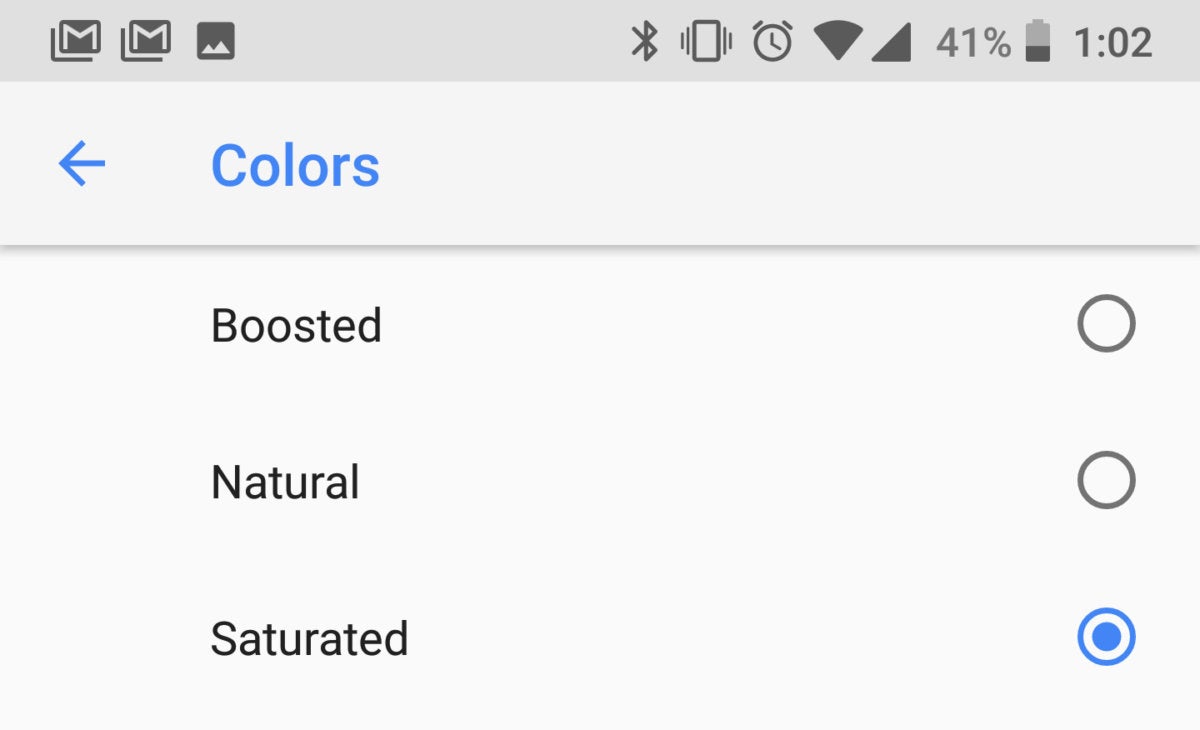This is a landscape-oriented screenshot captured from a smartphone, featuring a predominantly gray background. At the top, a darker gray bar spans horizontally across the screen, serving as a header. Within this bar, various icons are displayed from left to right: a Google Mail icon with a black envelope featuring a white "M", followed by a repeated icon, and a photo icon. Proceeding to the center-right side of the header are additional icons, including Bluetooth, a phone symbol set to vibrate (indicated by lines on either side), an alarm clock, a full Wi-Fi signal, a full network connection bar, the battery status showing 41% charge, a vertical battery icon with a black fill, and the time, displayed as 1:02.

Beneath the header, another horizontally aligned dark gray border separates the sections. This border includes a blue left arrow and the word "Colors" in blue. Below this, a lighter gray area encompasses three selectable options each accompanied by radio buttons to the right. The options listed are "Boosted," "Natural," and "Saturated." The "Saturated" option, located at the bottom, is currently selected. This is indicated by a blue line and a blue small circle in the radio button, set against a white background, signaling its active status.